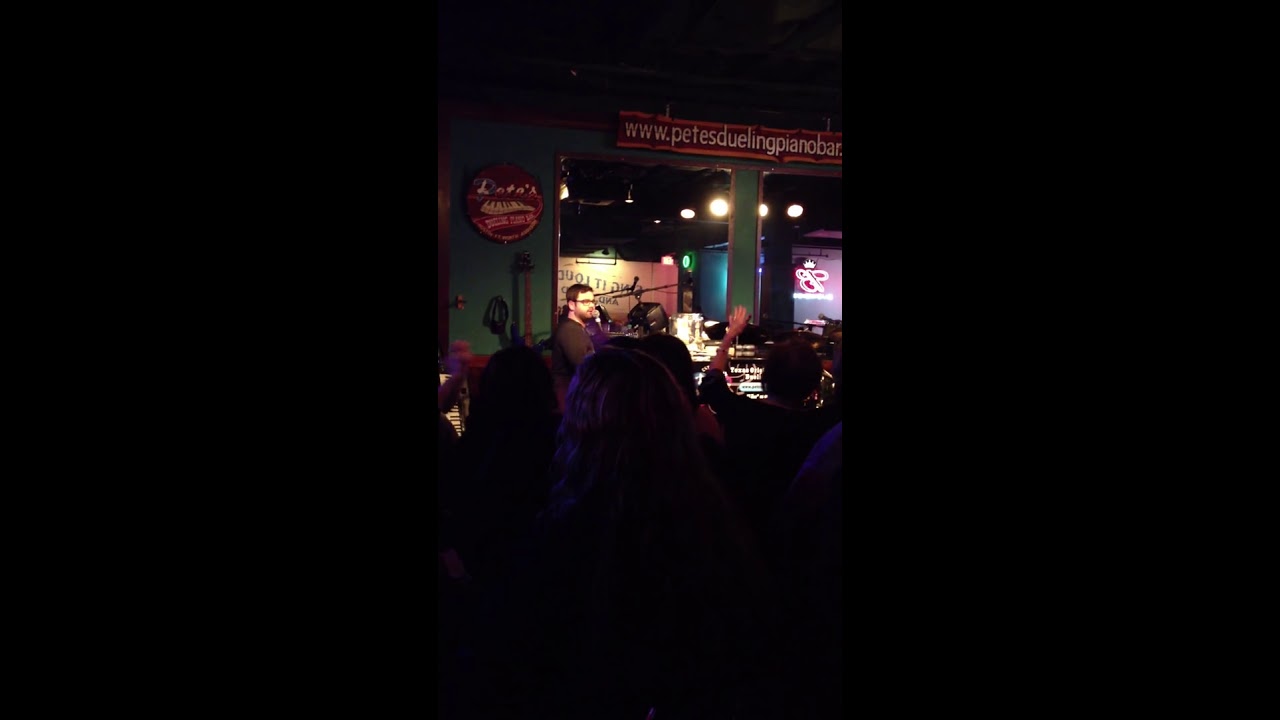In this detailed indoor photograph, a DJ, possibly part of a band, takes center stage, engaging with a lively crowd dancing and socializing in front of him. The setting appears to be a dimly lit bar or club, with various colored lights creating a vibrant atmosphere. The DJ, distinguishable by his dark brown, side-parted hair and glasses, wears a brown long-sleeve shirt. Behind him, a green wall adorned with a red board features a nearly legible website, www.PETESDUDUELINGPIANOBAR.com, written in white text. The ceiling is decorated with white lights, adding to the festive ambiance. Several people in the crowd, whose backs are mostly turned towards the camera, suggest an energetic, immersive musical experience. The color palette of the scene includes hues of yellow, orange, light brown, red, black, and dark green, heightened by the varying lighting. Whether daytime or nighttime remains unclear, though the presence of a roof confirms the indoor setting.